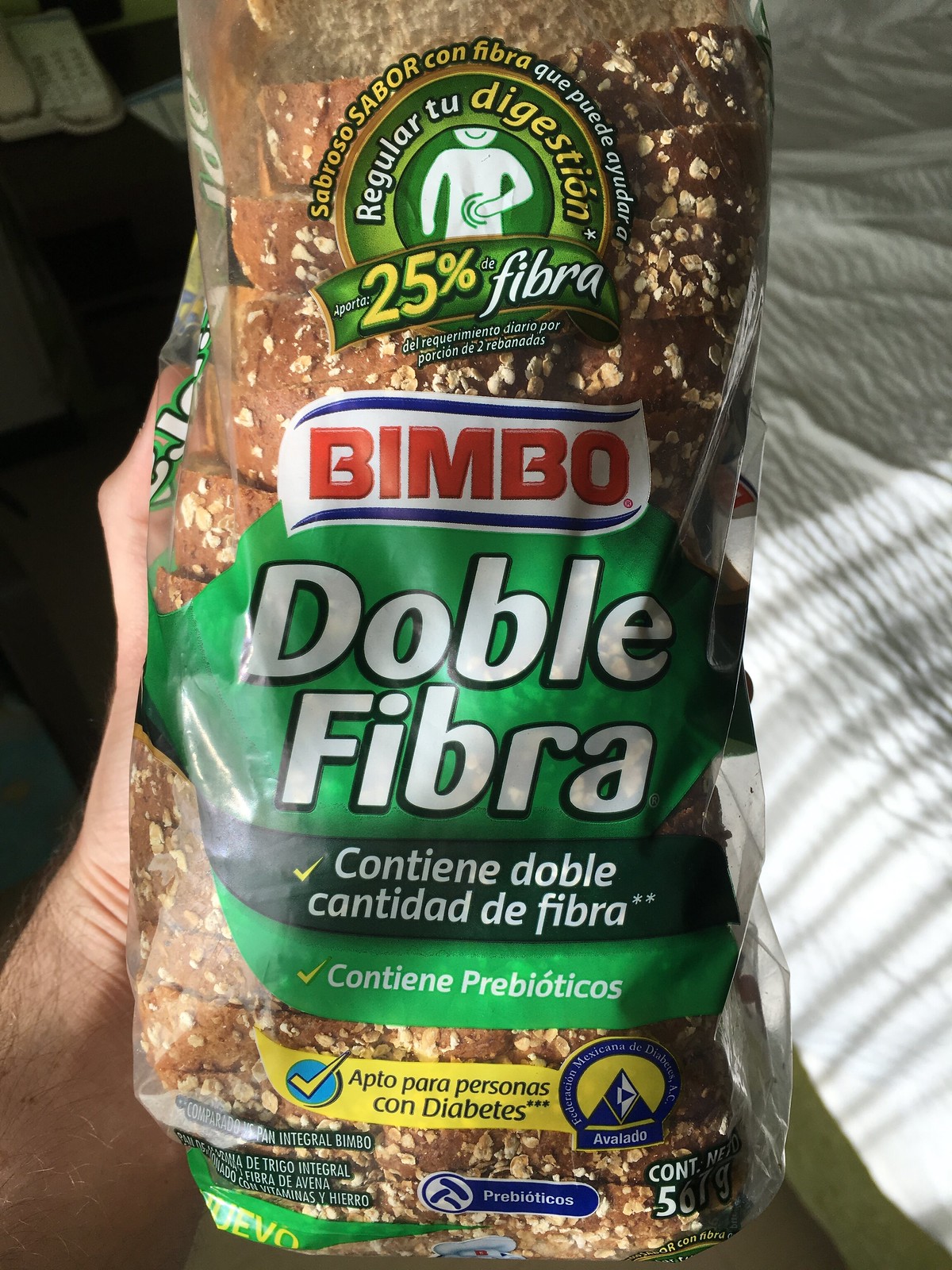In this photograph, a hand is prominently holding up a loaf of bread, labeled with a green and red, white, and blue packaging, marked with the brand name "Bimbo." The label on the bread, written in Spanish, reads "doble fibra," indicating that it is a high-fiber variety. The setting appears to be a bedroom, as evidenced by the presence of a white, slightly wrinkled sheet or comforter on a bed to the right side of the image. To the left, there is a wired house phone, adding a touch of domesticity to the scene. The hand holding the bread is positioned centrally, drawing attention to the product amidst the bedroom's casual, everyday surroundings.